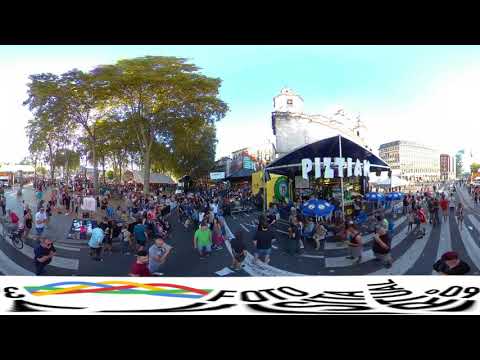This image captures a lively street festival in a city with the streets closed off to traffic. The scene is bustling with crowds of people in summer attire walking and exploring various booths lined along the streets, likely food stands. The main focal point of the photo features a tent with the word "PIZTIAN" or "PIZTIN" prominently displayed above it. Beneath this tent, there are numerous blue umbrellas adorned with white and yellow daisies, providing shade. The right side of the image shows trees casting shadows, suggesting it's a sunny day with some scattered white clouds. The photograph appears slightly distorted, possibly due to being taken with a VR or 360 camera. At the bottom, there's a colorful logo in blue, yellow, red, and green next to the word "photo" or "FOTO," though the text is somewhat stretched and difficult to decipher. Overall, the image vividly depicts a vibrant outdoor event with a cheerful, communal atmosphere.